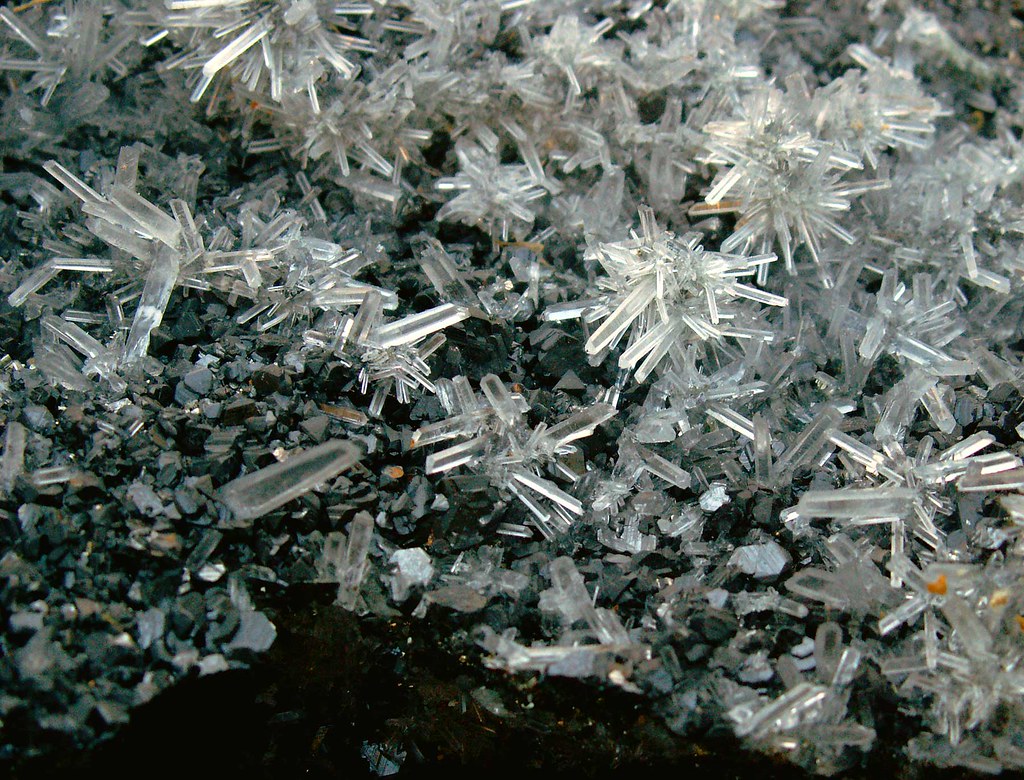The image captures an extreme close-up of crystallized formations, potentially resembling a geode or ice-covered pine needles. The composition spans from the top left to the bottom right, highlighting clusters of long, thin, glass-like crystalline structures that appear spiky and white or clear. These formations are densely packed, creating bowl-like assemblies across the screen, exposed to sunlight, which enhances their glistening appearance. Notably, there are some discolored areas, with an orange hue near the center and black, gravel-like structures towards the bottom, suggesting a contrasting underlying material or space resembling exposed rock. Towards the bottom left, a patch of unobscured greenery reveals green pine needles, providing a natural contrast to the icy or crystalline forms dominating the image. Overall, the photo meticulously details the intricate and mesmerizing patterns of these crystalline structures growing outward and interspersed with earthy elements.